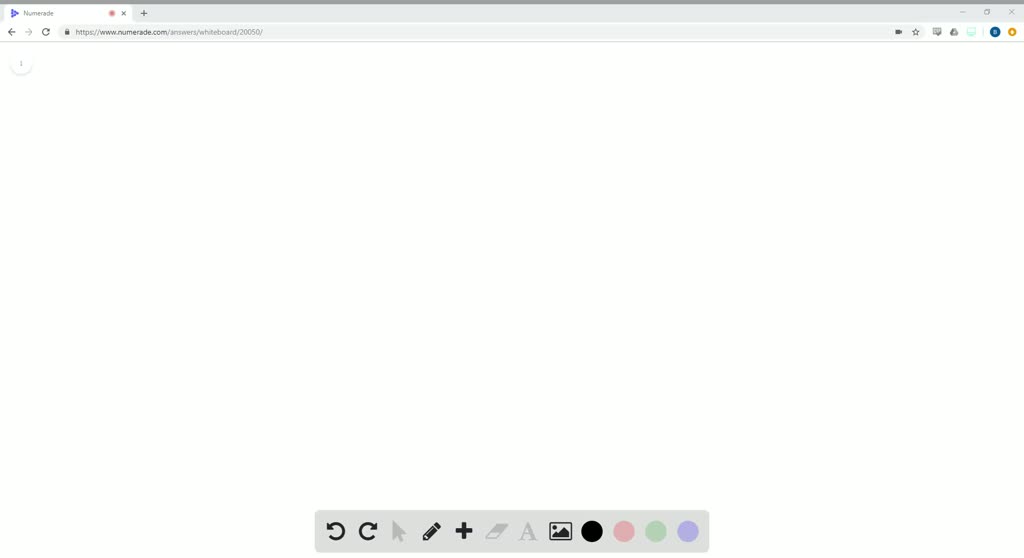The screenshot displays a web browser interface set against a white background. At the top of the interface, the browser's address bar contains a URL, while navigation buttons—including a left arrow, right arrow (grayed out), and a refresh button—are prominently shown. Additionally, a star icon and a white circle with two vertical dots are visible next to these buttons.

Below the address bar sits a gray toolbar containing various tools such as an undo button, a redo button, a gray down arrow, a pencil icon, and a plus icon, resembling an eraser. The workspace is divided into two sections: the top half in black or dark gray and the bottom half in white.

Also present in the interface is a gray capital letter "A", an image icon illustrating a mountain and sun with shading, and several colored circles—one black, one pink, one green, and one purple—add to the visual elements available on the screen.